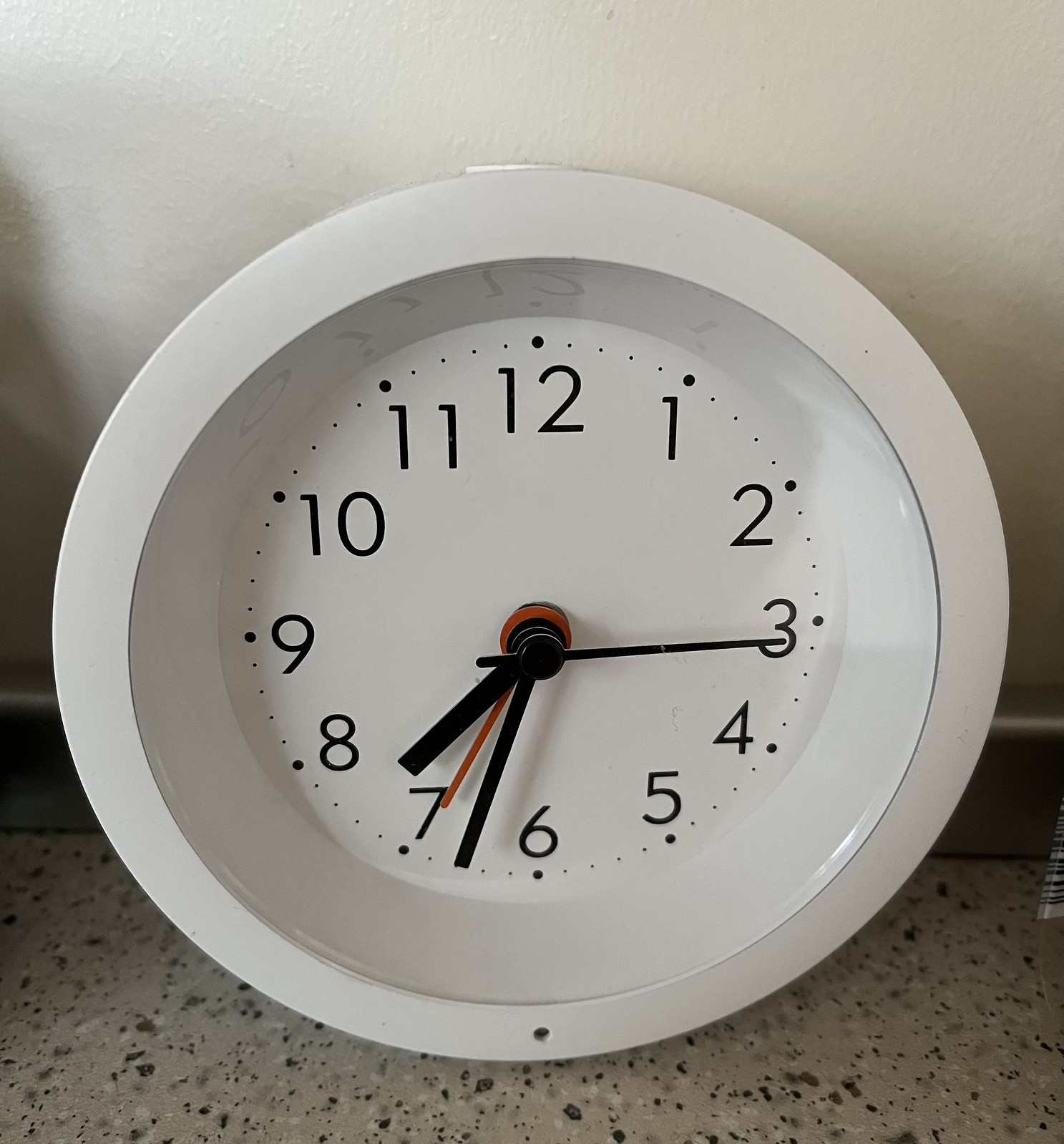The photograph depicts a circular white clock positioned against what seems to be either a floor or a countertop, with a plain white wall as its background. The clock's design is minimalist and entirely white, featuring a white border and face. Traditional black numbers from 1 to 12 mark the hours. The hour hand points just past the 7, and the minute hand is slightly beyond the 6, indicating the time is approximately 7:33. Additionally, the clock features a longer second hand positioned at the 3 and a distinctive red hand, making it more complex than a standard clock. Despite the extra hands, it maintains a conventional and unadorned appearance, blending seamlessly with its monochromatic environment.